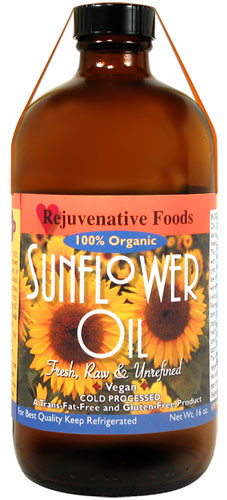The image depicts a bottle of sunflower oil set against a white background. The bottle, which has a dark brown medicinal appearance, features a black screw-on cap with a twist-off safety mechanism and a string or cord across the top. The label, which occupies most of the bottle, is adorned with vibrant sunflowers showcasing yellow petals and brown centers. At the top of the label, there's an artwork of a heart followed by the brand name "Rejuvenative Foods" and the description "100% Organic" in yellow letters within a blue oval. Additional text on the label reads "Sunflower Oil, Fresh, Raw, and Unrefined," emphasizing its organic nature. The product is also highlighted as vegan, cold-pressed, trans-fat-free, and gluten-free. The label advises keeping the oil refrigerated for best quality and indicates the net weight as 16oz.